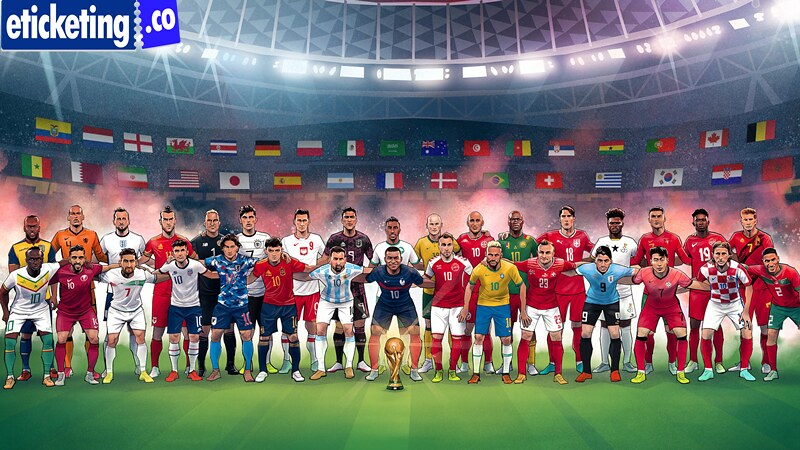This computer-generated image depicts an international soccer scene set in a covered stadium adorned with flags from various nations, capturing a World Cup celebration. It prominently features the text "eTicketing.co" in white on a blue background in the top left corner. The stadium is alive with a multitude of flags including those from Korea, Canada, Japan, America, Mexico, Wales, Australia, Switzerland, and Great Britain. Below these flags, on the lush green field, stand 32 soccer players arranged in two rows, each attired in unique jerseys that reflect their diverse national teams, with colors ranging from red and green to blue and black, to orange and purple. At the center of this vibrant assembly is a golden World Cup trophy, shining brightly. The central figure, a player wearing the number 10 jersey in blue, stands prominently in front of the trophy. The entire scene exudes a sense of unity and celebration, representing the global nature of the sport.